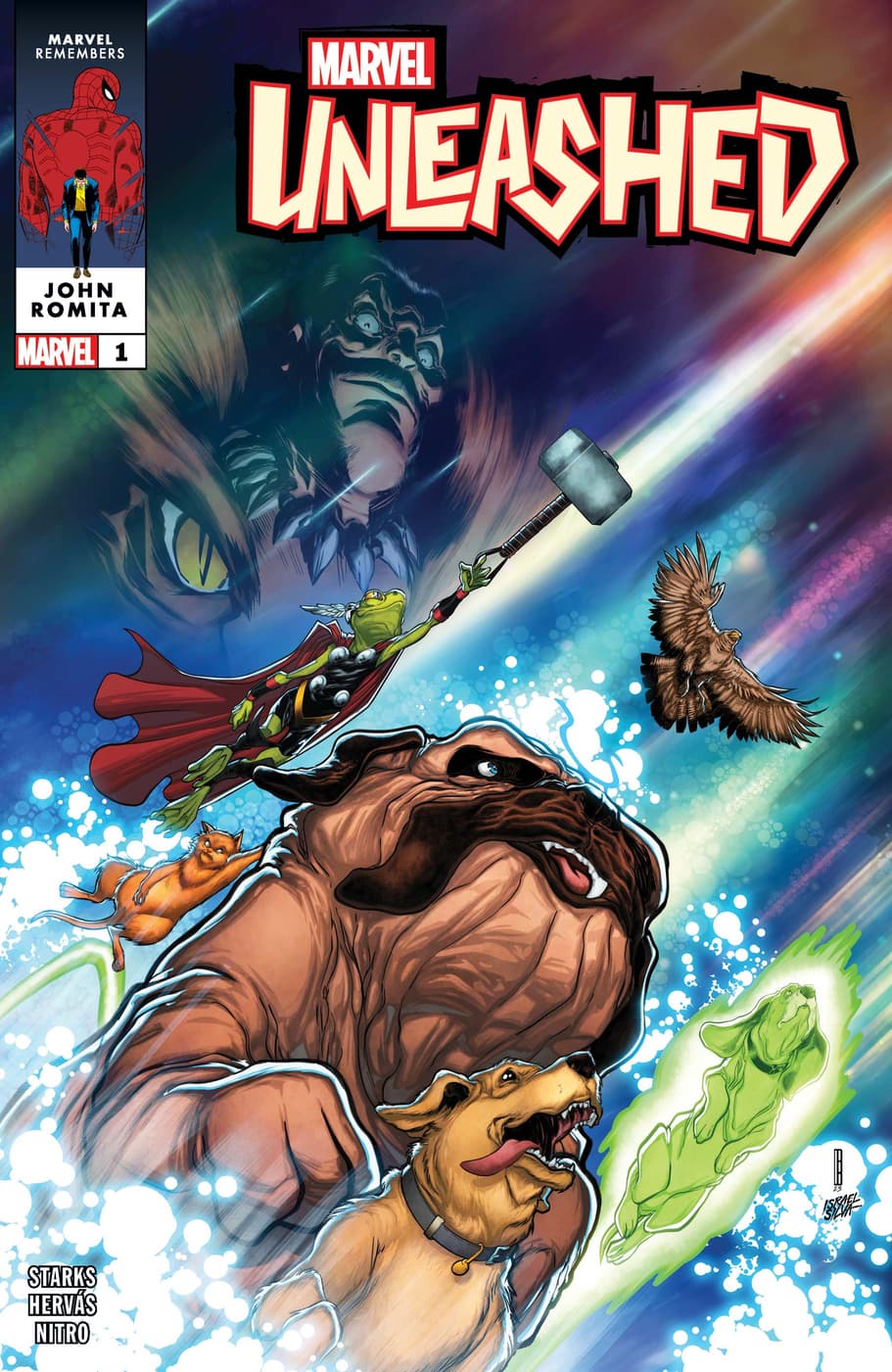The cover of the comic book "Marvel Unleashed" is a vivid color illustration set in portrait orientation. At the top, a red horizontal rectangle with white text reads "Marvel," and beneath it, white graffiti-style text bordered in black declares the title "UNLEASHED." Below this, the artwork features a dynamic scene: a large bulldog with loose skin and a determined expression is the central figure, depicted from above with its fangs bared and one paw raised. Directly below, a golden retriever with its tongue hanging out flies alongside the bulldog, looking happy and eager. A smaller, golden-colored dog and a cat clinging to the bulldog's back are also part of the ensemble.

Surrounding these main characters are other flying creatures: a frog dressed in armor with a winged helmet and holding a hammer, a brown eagle, and a green futuristic-looking dog. The backdrop is a dark blue sky streaked with colors, suggesting they are soaring through space or a similarly vast expanse.

On the upper left of the cover, a sinister witch-like figure with long hair looms in the shadows, frowning down at the scene. Just below her is a vertical panel labeled "Marvel remembers," followed by a white horizontal rectangle that reads "John Romita," another red rectangle with the Marvel logo, and a white box with the number "1" in black text, indicating this is the first issue. The detailed illustration captures a sense of action and adventure, setting the tone for the comic's storyline.